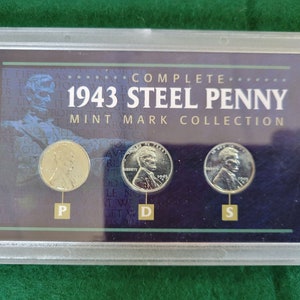The image showcases a meticulously framed, complete 1943 steel penny mint mark collection, positioned against a rich, dark jade green background with a marble-like texture. The collection is encased in a light gray wooden frame with a clear plastic cover, reflecting hints of a smartphone held up by the photographer. Centered within the frame is a dark blue background featuring an image of the Abraham Lincoln Memorial statue, and across the top in bold white letters, it reads "Complete 1943 Steel Penny". Below this, in a slightly smaller yellow print, it states "Mint Mark Collection". The collection consists of three shiny steel pennies, each distinctly labeled: the first on the left marked 'P', the middle one marked 'D', and the one on the right marked 'S'. The 'P' penny appears particularly bright and golden, potentially due to lighting. The artwork also includes subtle lettering across the background, enhancing the historical and commemorative essence of this coin collection.